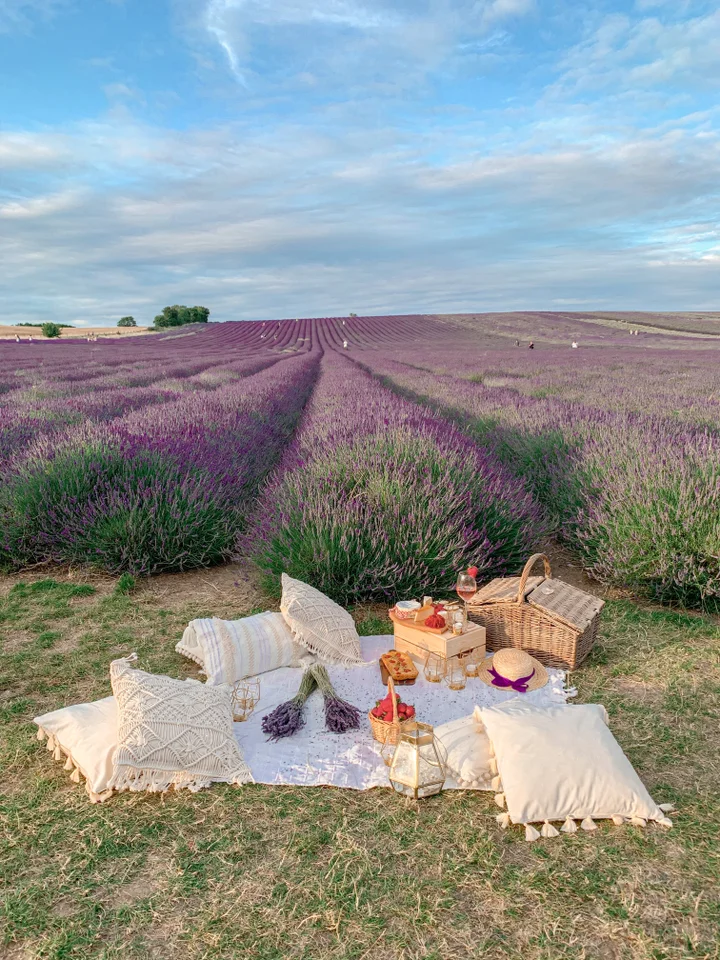The image captures an idyllic outdoor picnic set in a vast field of tall grass which transitions from green at the bottom to purple at the top, resembling lavender. This expansive field stretches far into the distance, emphasizing its large size. Situated at the bottom portion of the image, the picnic setup features a white blanket adorned with beige pillows, some with tassels and varied textures, including knit and cotton, and some striped. Arranged on the blanket is a classic woven picnic basket, a light wood crate with a cheese board, assorted cheeses, glasses, candles, and a sun hat with a purple bow. There are also baskets, one filled with strawberries, and two bouquets of flowers that blend seamlessly with the surrounding purple and green grass. In the backdrop, a clear, bright blue sky with white clouds adds to the serene ambiance of the scene. The overall image is vibrant and detailed, capturing the bright and clear setting with excellent clarity. The horizon shows some brown land and trees, providing a natural frame to the vertical furrows of the field that extend towards it.